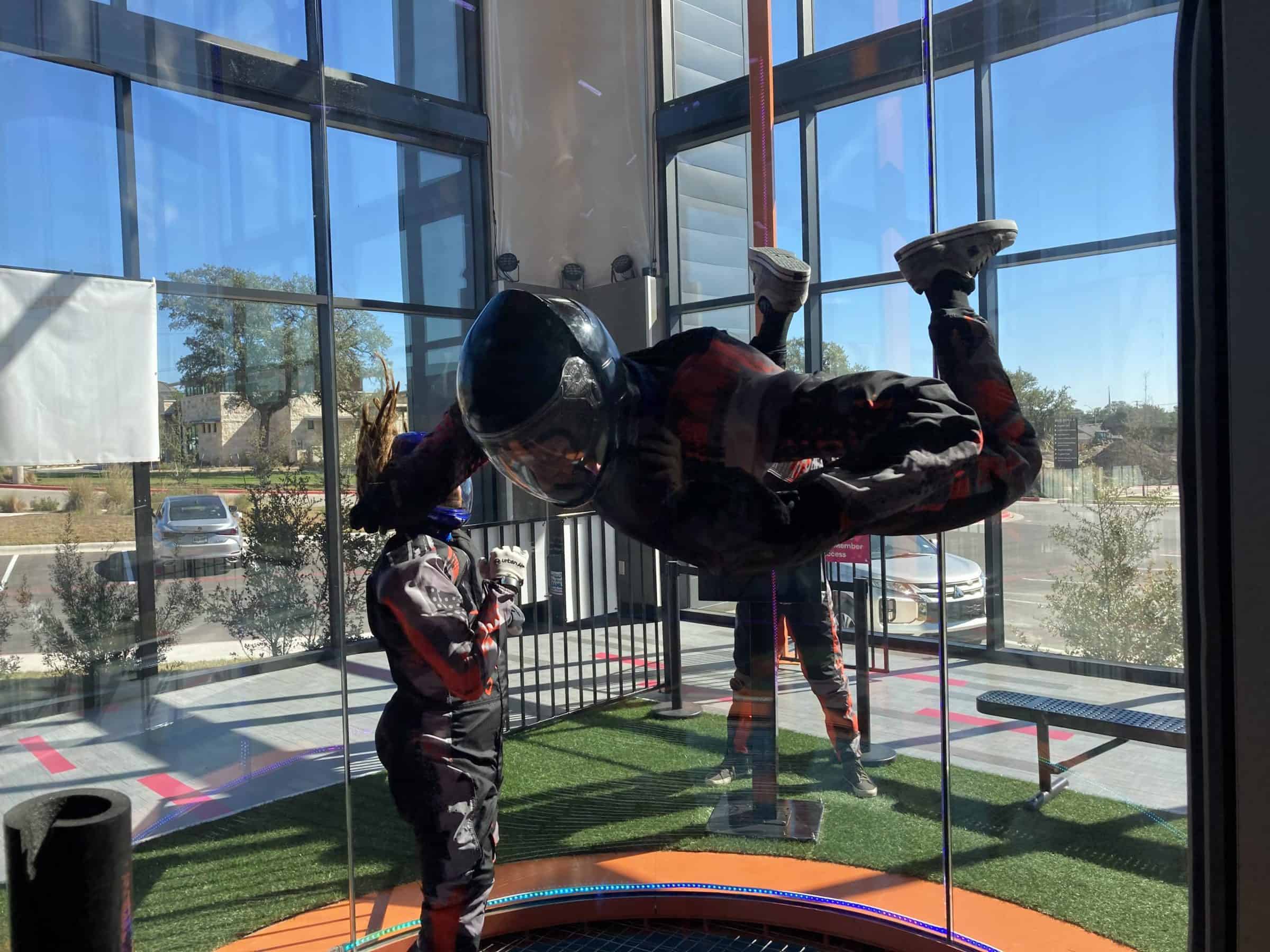This detailed photograph captures the exhilarating experience of indoor skydiving inside a large glass-encased vertical wind tunnel. At the center of the image, a person in a dark skydiving suit with red accents on the shoulders and hands, along with a protective helmet, is seen floating mid-air, enjoying the sensation of freefall as the updraft of powerful airflow simulates the skydiving experience. To the side, a second individual dressed identically stands on the floor of the wind tunnel, likely awaiting their turn or assisting. Outside the transparent cylindrical enclosure, yet another person in similar equipment observes the activity. The scene takes place within a spacious building characterized by its floor-to-ceiling glass walls that offer a clear view of the outside. In the background, a parking lot stretches into the distance with several white and silver cars, flanked by a tan building and a cluster of trees to the right, all under the bright daylight. The image vividly captures the dynamic and gravity-defying experience of indoor skydiving in a modern, light-filled facility.